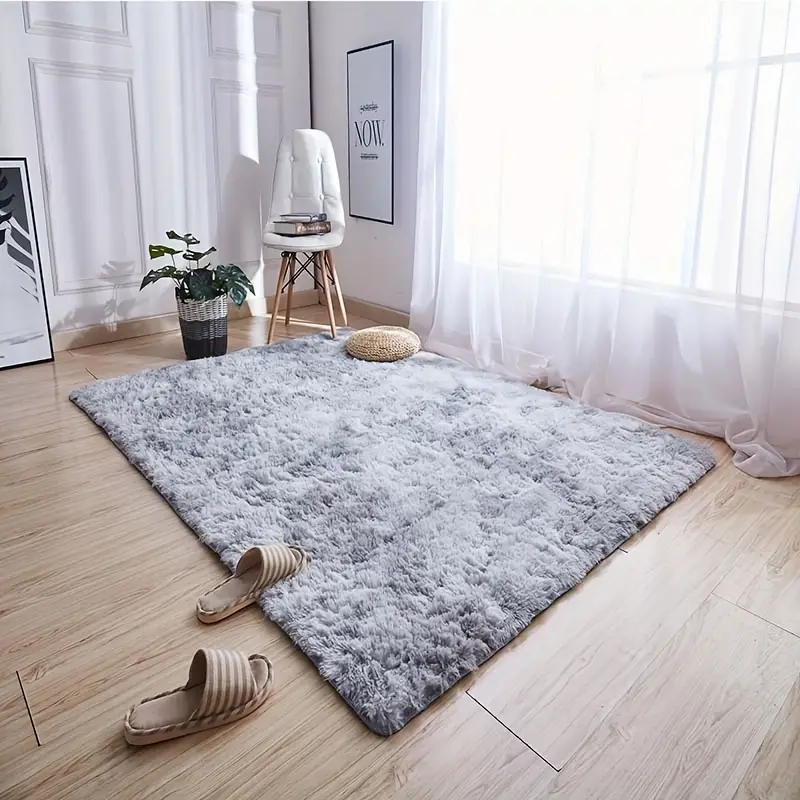This interior shot captures a cozy corner of a room adorned with light-colored wood plank flooring. Sunlight pours in through a large window on the right, draped with a sheer white curtain. Below the window, a furry gray rectangular rug lays on the floor, partially covering a pair of tan and brown striped slippers. A small round cushion rests near the edge of the rug. In the corner, a sleek white chair with wooden legs supports a pile of books. Adjacent to the chair, a gray, black, and white planter houses a small green plant. The white walls feature wainscoting on the left side, where a large black-framed poster bearing the word "now" leans casually. This serene space is complemented by the airy ambiance created by natural light and simple, yet thoughtful decor elements.